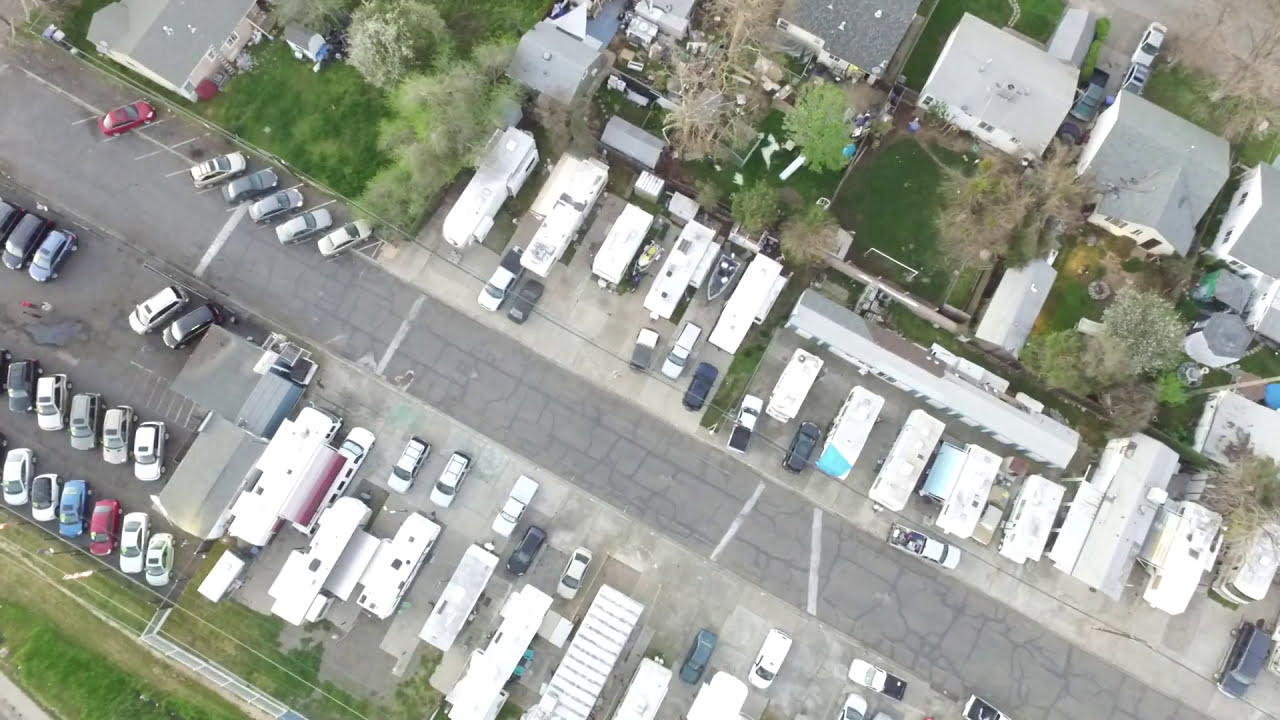The image is a detailed, color, aerial view of a neighborhood, captured in landscape orientation from a drone during the daytime. At the center of the composition is a prominent gray paved street running diagonally from the top left corner to the bottom right corner. Flanking the street on both sides is a row of approximately 20 white RVs and motorhomes, along with other parked vehicles, some of which include boats beside them. On the left side, about 12 to 15 cars are lined up, while intermittent green trees are scattered throughout the vicinity, with lush grass visible below and beside the fenced areas separating the RVs. In contrast, the right side of the image features a couple of two-story houses and some smaller single-family detached homes towards the top of the image, characterized by their mostly gray roofs. The backyards of these houses show a mix of greenery, trees, and fences, which delineate the properties from the roadway. The scene showcases a realistic and representational photographic style, highlighting the ordered layout and natural elements present in this motorhome-dominated neighborhood.